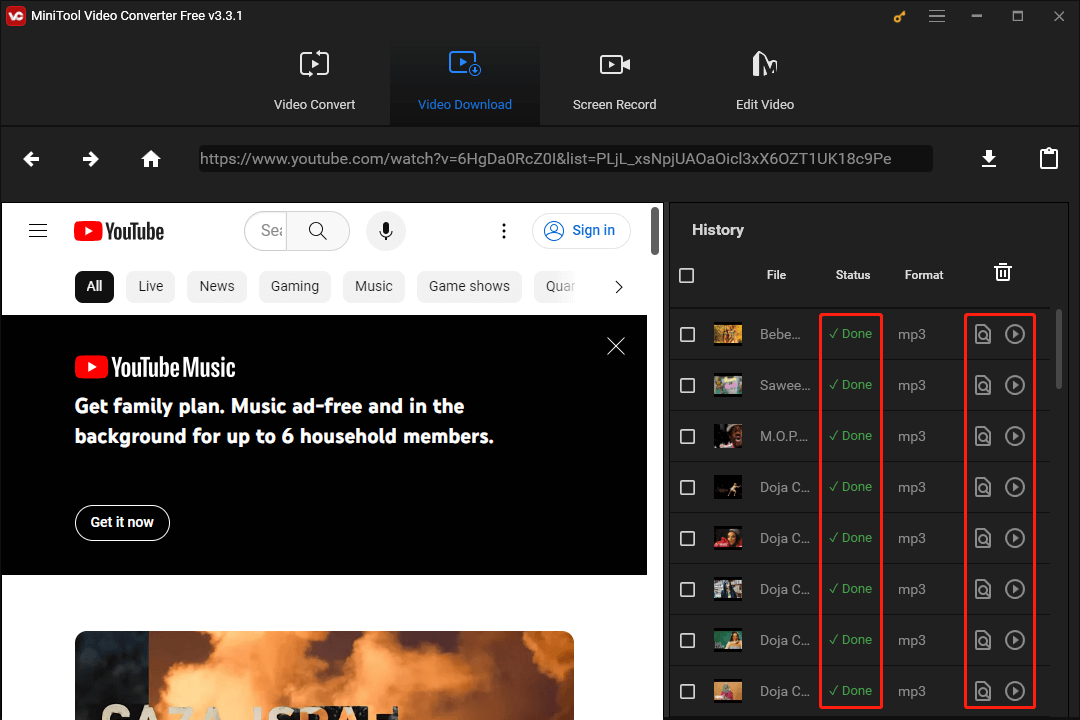The image showcases a web page belonging to a YouTube downloader application called MiniTool Video Converter Free Version 3.3.1. At the top of the page, the header prominently displays the software name along with navigation buttons, the "Video Download" button being highlighted. Below the header, a YouTube Music advertisement is visible. This advertisement encourages users to get a Family Plan, offering ad-free music for up to six household members and features a "Get It Now" call-to-action button. The main section of the page is focused on the download history, which features various downloaded videos marked with a red outline, indicating successful downloads. Additionally, a partial image of a cloudy, yellow-toned sky is visible beneath the download history, possibly related to one of the downloaded videos.